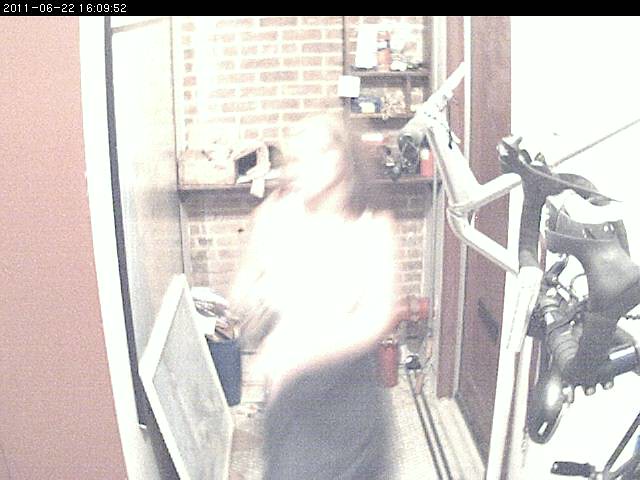A blurry photograph captures the silhouette of a person, potentially a woman, dressed in a white top and a black skirt standing in a narrow, cluttered space. The backdrop reveals a brick wall adorned with shelves, one of which holds a box. The corner is densely packed with various items, resembling a chaotic assortment of junk. Prominently visible is a red pipe that emerges from the floor and extends into the wall on the right side. Among the clutter, there is a picture frame and a blue tote filled with papers and miscellaneous objects. To the right of the woman, in the foreground, stands a piece of black and metal machinery, adding to the overall disarray of the scene.